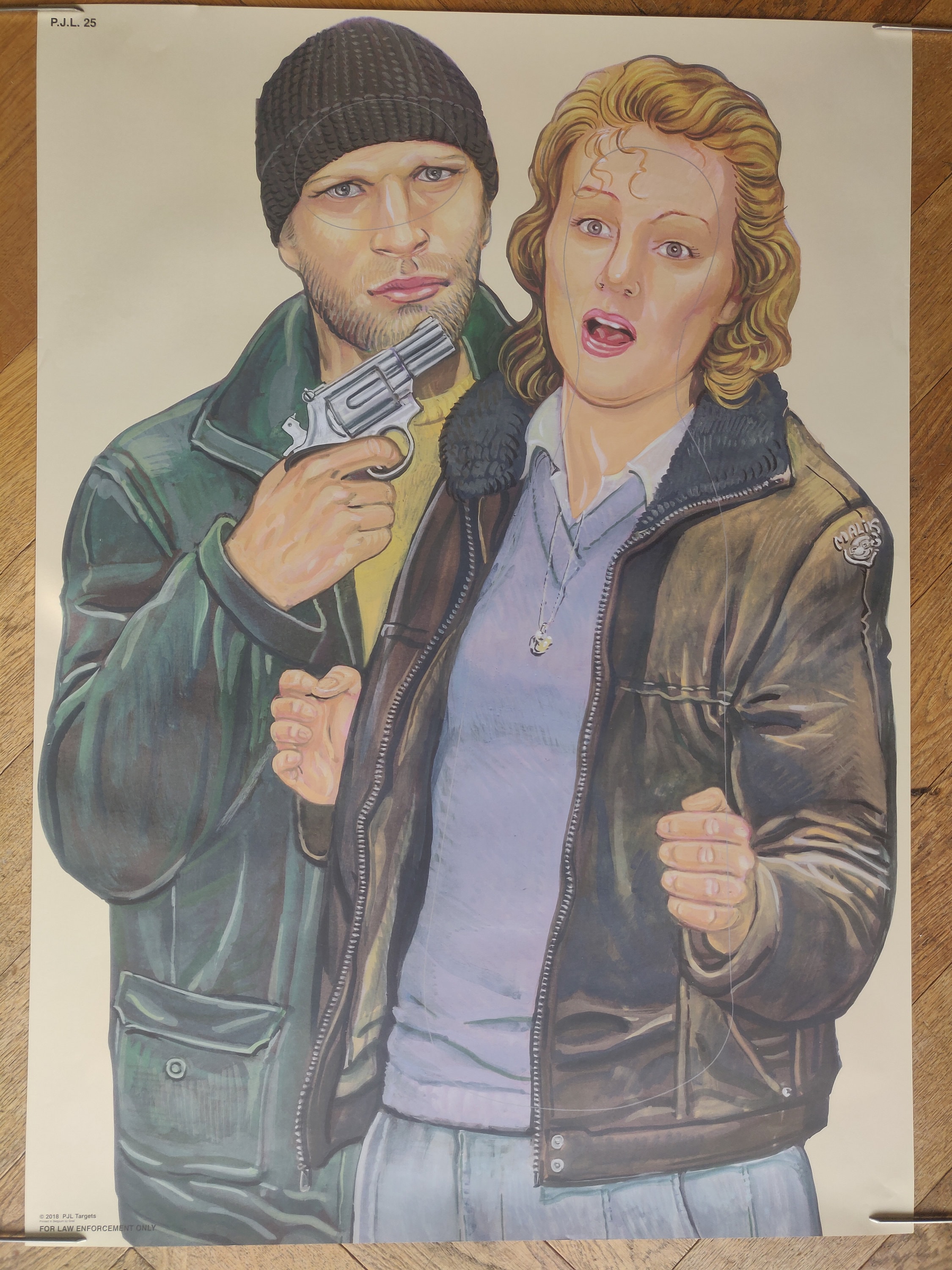This is a detailed, hand-drawn artwork set within a wooden frame, depicting a tense scenario between a man and a woman. The man, positioned to the left, is wearing a black beanie and sports a beard without a mustache. Clad in a green jacket over a yellow shirt, he is holding a cocked revolver aimed directly at the woman's head, his finger on the trigger. The man’s intent expression contrasts with the woman's evident distress. 

The woman, standing on the right, has short, curly blonde hair. She is donned in a brown leather bomber jacket with a fur collar and a noticeable emblem on the shoulder reading "Mally's." Underneath her jacket, she wears a light purple or blue sweater revealing a white collared shirt beneath, and around her neck, she sports a silver necklace with a pendant. She appears to be gasping or calling for help, her hands lowered to her sides.

Background details indicate that this image likely serves as a shooting target, with specific marks for aiming, including a circle around the man's eyes and a demarcated outline on the woman's figure. Notably, in the top left corner of the drawing are the initials "PJL 25," and at the bottom, it states "For law enforcement only 2018 PJL targets." The entire scene is set against a stark white background, emphasizing the dramatic interplay between the characters.